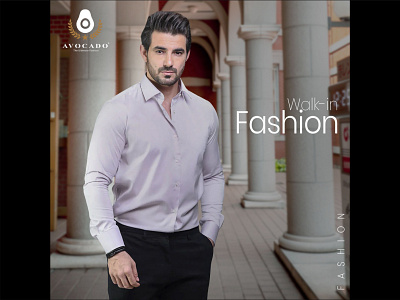This image is a detailed photograph from a fashion magazine. The top left corner features a banner with an avocado symbol and the text "Avocado" below it. The main headline reads "Walk-in Fashion," with "fashion" in larger, bold white text underneath. The spotlight of the image is on a well-dressed man posing elegantly between tall white columns, of which seven are visible — five to his right and two to his left. He is wearing a light-colored shirt that appears white or possibly a very light purple/pink, paired with black pants. The man has a neatly groomed short beard and mustache, and his dark black hair is styled upward. One hand is placed in his pocket while the other rests by his side, and he gazes directly at the camera. Behind him, a brown wall contrasts with the columns, adding depth to the scene. Overall, the setting appears to be in front of a refined building, possibly under an archway.